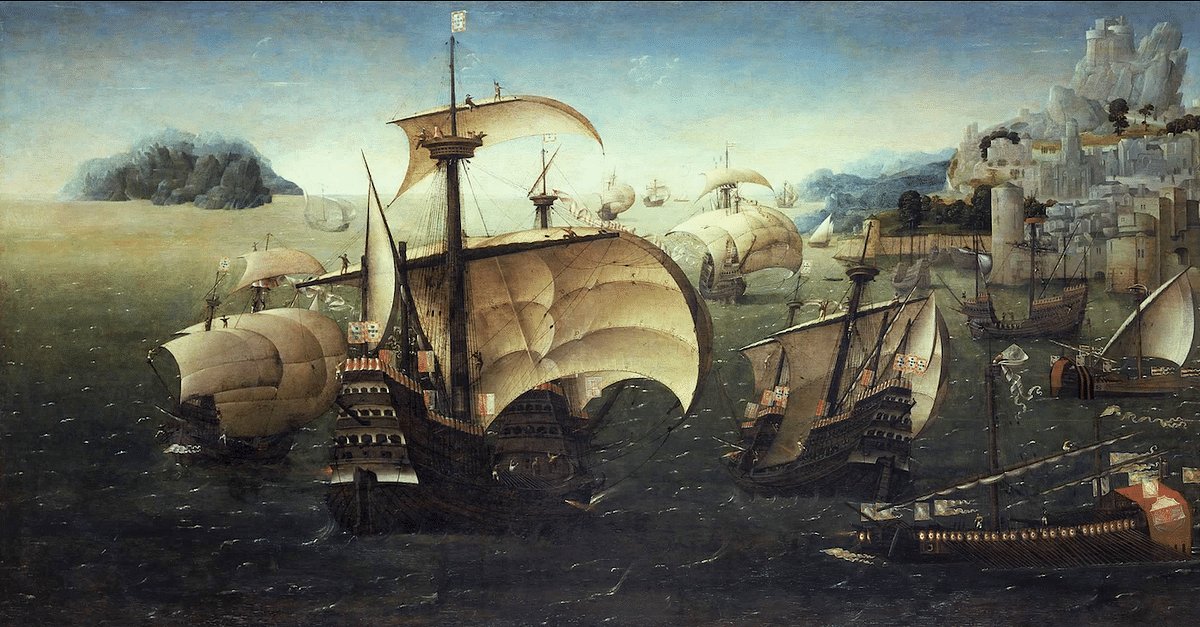The painting is a dark, atmospheric scene of a tumultuous ocean with dark green, choppy waves, and white caps under a sky scattered with clouds. At the center of the image, slightly to the left, a large, historic wooden ship dominates, its tall masts topped with tan-white, cream-colored sails billowing in the wind. There are two people visible high up on the top sail, well above the crow's nest, while a flag flutters at the pinnacle of the mast. Surrounding the main ship are several smaller vessels with similar designs, including two particularly notable ones—one small ship directly to its right and another just above it.

In the background, on the left horizon, there is an ambiguous large grayish formation which might be a rock or a dark cloud. To the right, the shoreline is visible where a fortified city, with its white cream-colored buildings and castle-like structures atop a hillside, stands prominently. The city features a wall running along the land and larger white rocks or rounded ramparts crowning the top of the hill. The cityscape and crowd of ships together convey the painting's dynamic and historical essence.